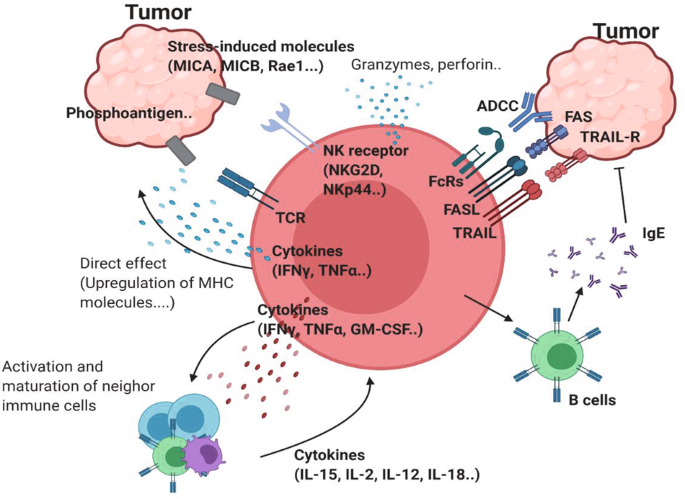The illustration is a detailed diagram, likely from a medical textbook, depicting the interaction between tumors and the immune system. At the top left and top right corners, the term "tumor" is labeled, each representing a tumor-like structure with a fleshy, cloud-like appearance. The top left tumor includes labels such as "stress-induced molecules" with specific markers like MICA, MICB, and RAE-1, connected through gray arrows pointing towards a central cell.

Beneath this fleshy tumor-like blob is the term "phosphoantigen," surrounded by arrows pointing towards a central circle, which appears to represent an immune cell. This central cell is illustrated in darker pink and contains numerous labels, including "granzymes," "perforin," "NK receptors," "TCRs," and "cytokines." Beyond this central cell, more arrows point towards another tumor-like structure on the right, indicating further molecular interactions and immune responses.

The right-side tumor is similarly labeled with terms such as "ADCC," with green and blue electrochemical shapes surrounding it. The diagram also includes sections on the "activation and maturation of neighbor immune cells" and the "upregulation of MHC molecules.” Various immune cells, including blue and green B cells, are depicted, showing interactions with antigens like IgE.

Overall, the illustration effectively details the complex interplay between tumors and the immune system, highlighting specific molecules and processes involved in the immune response to tumor cells.